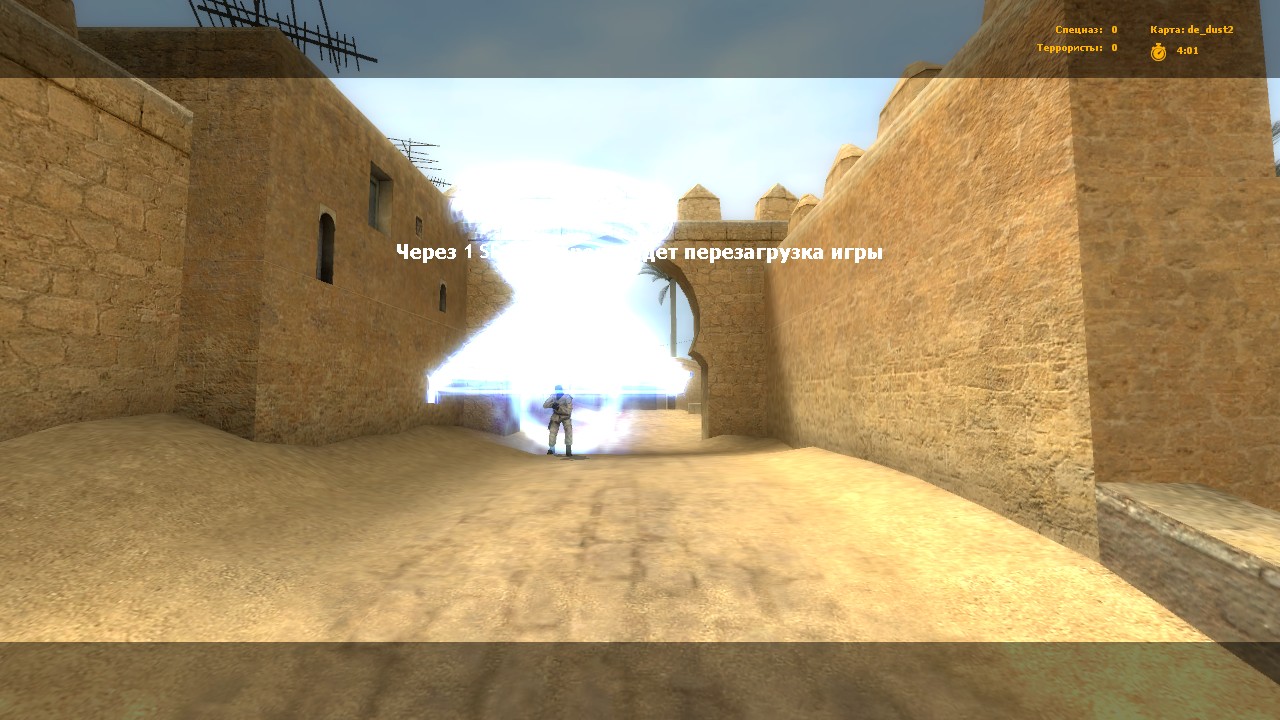A detailed caption for the image could be:

"A captivating screenshot from a video game features a prominent character in a white outfit emerging from a radiant blue light at the center. The upper and lower edges of the image are bordered by gray, translucent bands, framing the scene. The backdrop reveals a sandy-colored road leading into a stone-walled area, where the walls display a rich, yellowish-orange hue and stand about four times the height of the character. These walls include numerous window-like cutouts. The environment exudes a desert-like atmosphere with intricate architectural elements. Overlaying the image is white text in a foreign language, while the upper right corner also contains orange text in another language."